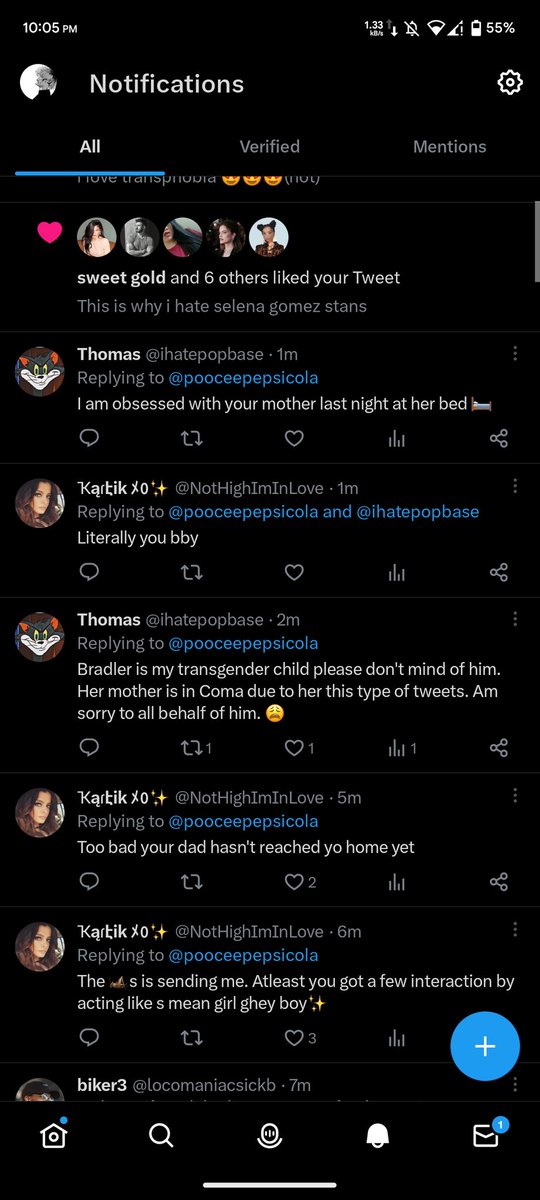In this image, the screen displays a social media notification page against a solid black background. At the top of the screen, the current time is shown as 10:05, accompanied by a battery indicator at 56%. Below this, a circular profile icon appears next to the word "Notifications". To the right, there is a small white cog icon, representing the settings button.

The notification section is categorized into "All", "Verified", and "Mentions", with "All" being underlined in blue, indicating it's the active tab. Beneath these tabs, a notification indicates that "sweet_gold and five others" liked a tweet by the user.

Several tweets are displayed, beginning with a controversial tweet by Thomas that reads, "I am obsessed with your mother last night at her bed." Further responses include:

1. A tweet from K: "XO literally you baby."
2. Another reply from Thomas: "Bradley is my transgender child, please don't mind of him. Her mother is in a coma due to her. This type of tweets I am sorry to all on behalf of him." It ends with a frowny face emoticon.
3. K responds: "Too bad for you dad hasn't reached yo home yet."
4. Another tweet from K: "Is this something new? At least you get a few interactions by acting ill or acting like a mean girl or gay boy."

To the right side of the screen, a blue circle with a plus sign is evident. At the bottom, various navigation icons are present: "Home" with a blue dot, a magnifying glass for search, a circle with a line under it to represent profile, a bell for notifications, and a mail icon with a blue circle and the number 1, indicating an unread message. A white line runs across the bottom, separating these icons from the rest of the content.